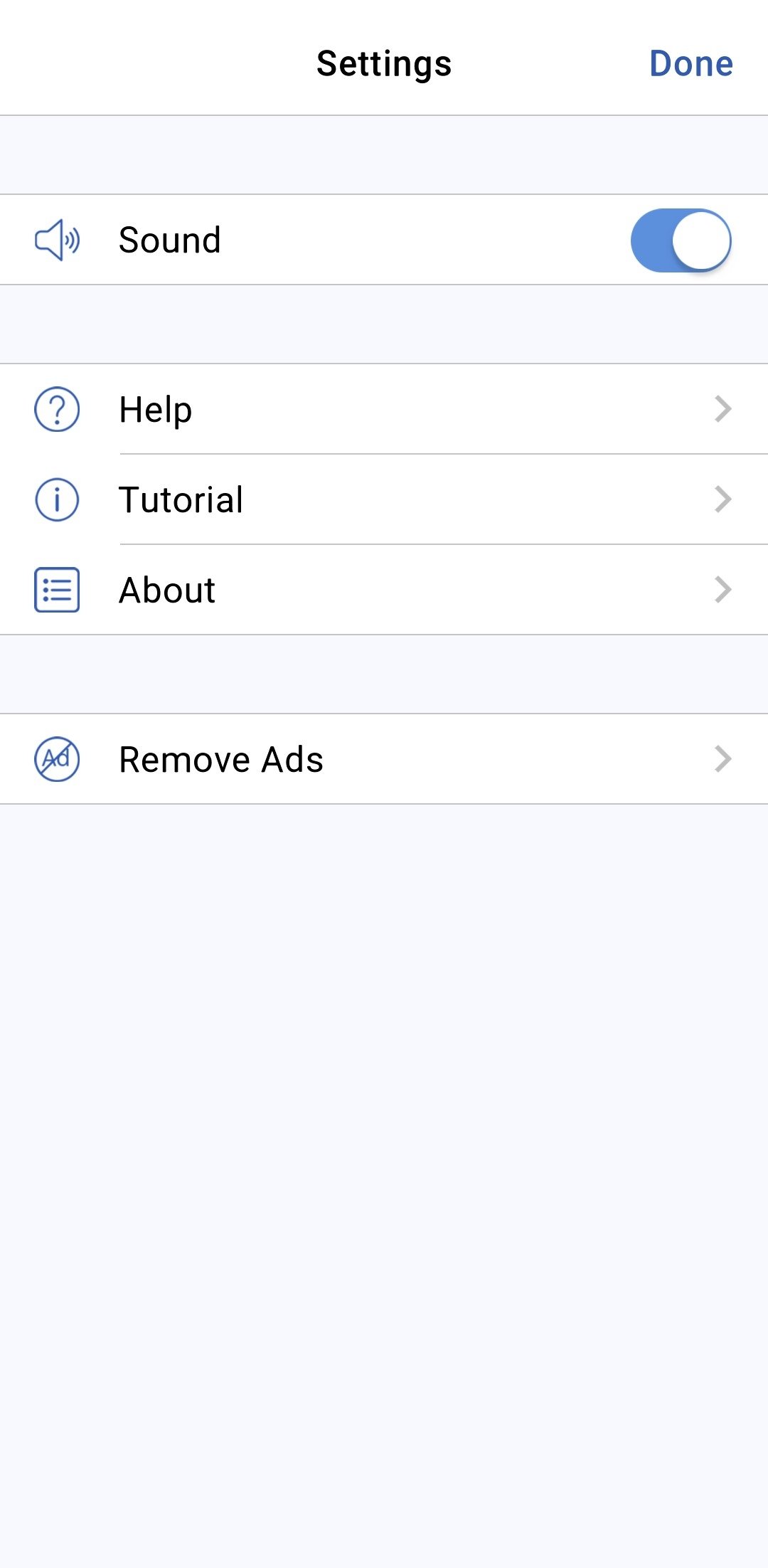The image depicts a detailed section of a program or app displayed in portrait orientation. The background gradually transitions from a pure white at the top to a very pale blue in the bottom half. The screen is organized into several horizontal rows, each delineated by thin gray lines.

At the very top, centered on the white background, the word "Settings" is displayed in bold black letters. In the top right corner, "Done" appears in blue, signifying a button to exit the settings menu. Below this, a horizontal pale blue bar serves as a separator. 

The first interactive row is white and labeled "Sound." On the left is an icon of a speaker emitting sound waves. To the right, there is an on/off toggle switch resembling a blue oval with a white circle, which is currently toggled to the "on" position. 

Next, there is a plain blue bar, followed by another white row labeled "Help." This row features a question mark inside a circle icon and an arrow on the far right, indicating a menu that can be expanded for further options.

The next row is labeled "Tutorial," featuring an information icon inside a circle, followed by another white row labeled "About" with an icon resembling a document.

Another pale blue bar follows, beneath which is a white row labeled "Remove Ads." This row includes an icon of a circle labeled "Ad" with a strikethrough and an expandable arrow on the right.

The remainder of the screen is filled with the very pale blue color, providing a soft background contrast to the various interactive elements above.